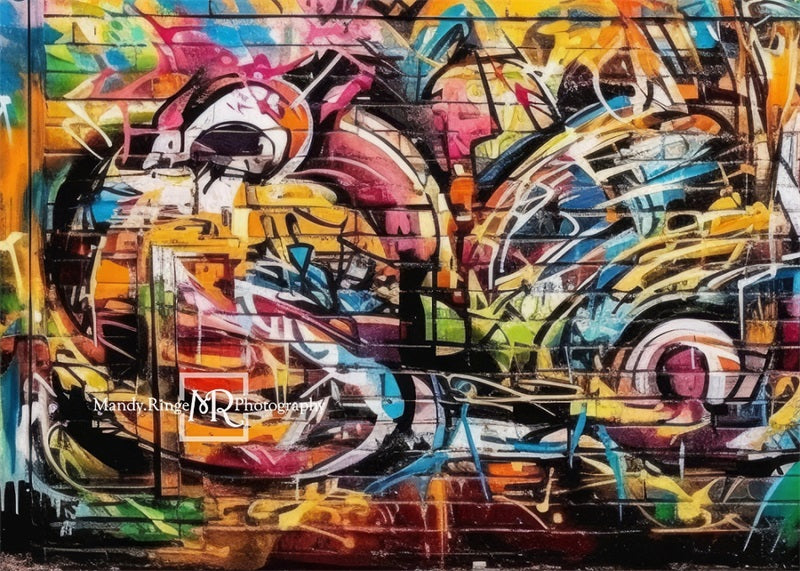This photograph captures a brick wall almost entirely obscured by vibrant graffiti. The wall, signed with "Banny Ringe Photography" in a white cursive watermark, is a chaotic canvas of street art layers, where a possible underlying mural is buried beneath random tags and streaks of spray paint. Dominant colors like pink, blue, orange, yellow, green, white, electric blue, purple, and black intermingle, with round shapes and splashes suggesting various abstract elements—almost forming enigmatic figures, possibly eyes or a motorcycle profile. Despite the disorderly overlay, the eclectic mix of colors and forms conveys a passionate expression of the artists involved.